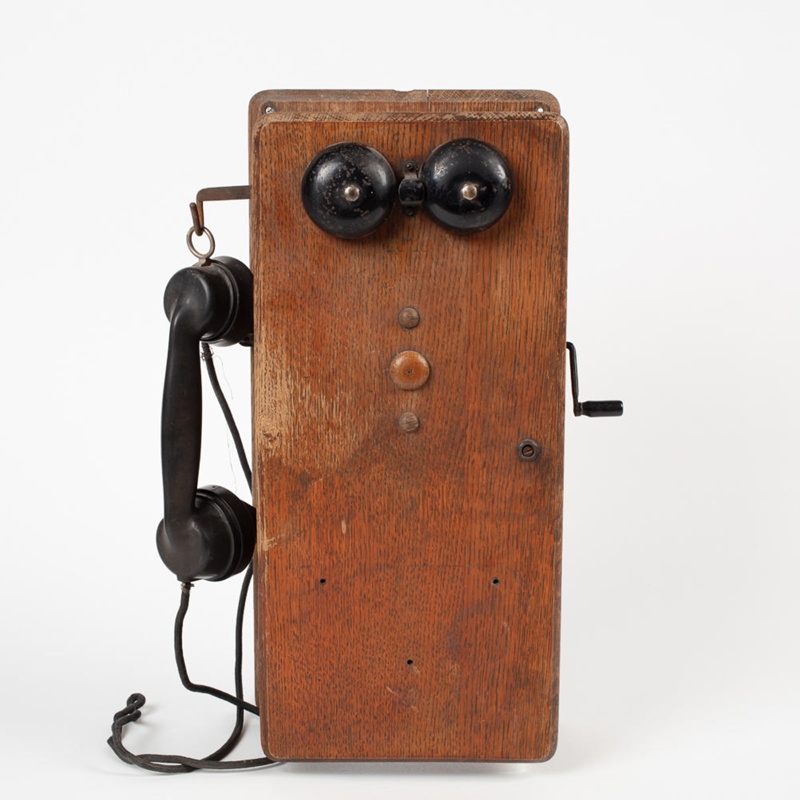This color photograph features an antique, wind-up telephone set against a white background. The telephone, centrally positioned in the image, is constructed from worn, light brown wood and has a vertical, rectangular shape. At the top of the telephone are two round, black bells that almost resemble eyes, each fastened with silver screws and connected by a rod. Just below the bells are three small, wood-like buttons. 

On the left side of the telephone, a black handset with a wire hangs from a hook, its cord extending from the top part of the handset to the telephone itself. The handset, which combines both the listening and speaking functions, dangles beside the wooden box. On the right side of the telephone, there is a distinctively attached handle or crank, used for making phone calls. The worn appearance of the wood accentuates the telephone’s antiquity and historical significance.